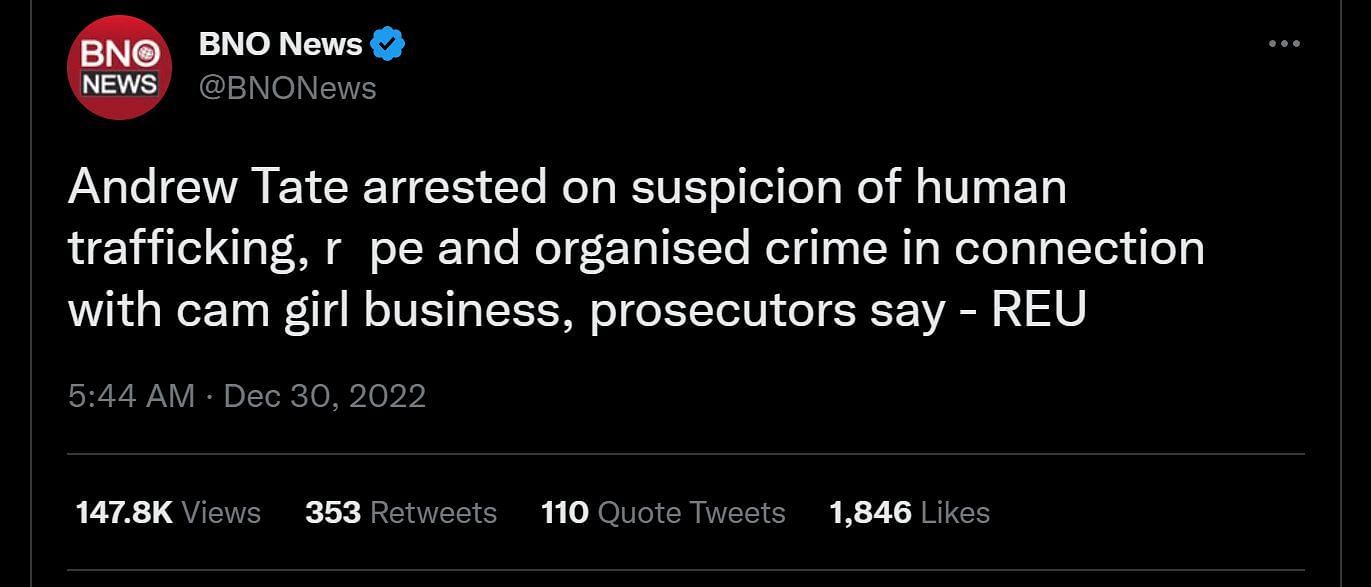**Screenshot from Twitter/X: BNO News Reports on Andrew Tate's Arrest**

The image captures a screenshot from BNO News' Twitter/X feed, displaying a tweet on a completely black background. 

- **Top Left Corner:** A distinctive red circle with the capital letters "BN" and a small logo within it, positioned above the text "News" in white on a black background.
- **To the Right of the Circle:** The full name "BNO News" in white text is prominently displayed. Just beside it, a blue circle with a black check mark signifies the verified status of the account.
- **Beneath This Text:** "BNO News" is written in lighter gray text followed by the handle "@BNO News."

**Main Tweet Text:**
- Larger white text announces: "Andrew Tate arrested on suspicion of human trafficking, rape, and organized crime in connection with cam girl business, prosecutors say - REU."

**Timestamp and Interaction Stats:**
- In smaller gray text, the timestamp reads: "5:44 a.m. · December 30, 2022," followed by a thin gray horizontal line running across the bottom of the tweet.
- Below the line, interaction statistics are presented:
  - "147.8K" in bold white denotes views.
  - "353" in bold white indicates retweets.
  - "110" in bold white signifies quote tweets.
  - "1846" in bold white shows likes.

The overall presentation and detailed elements convey the gravity of the news while maintaining a clear and organized layout for viewers.